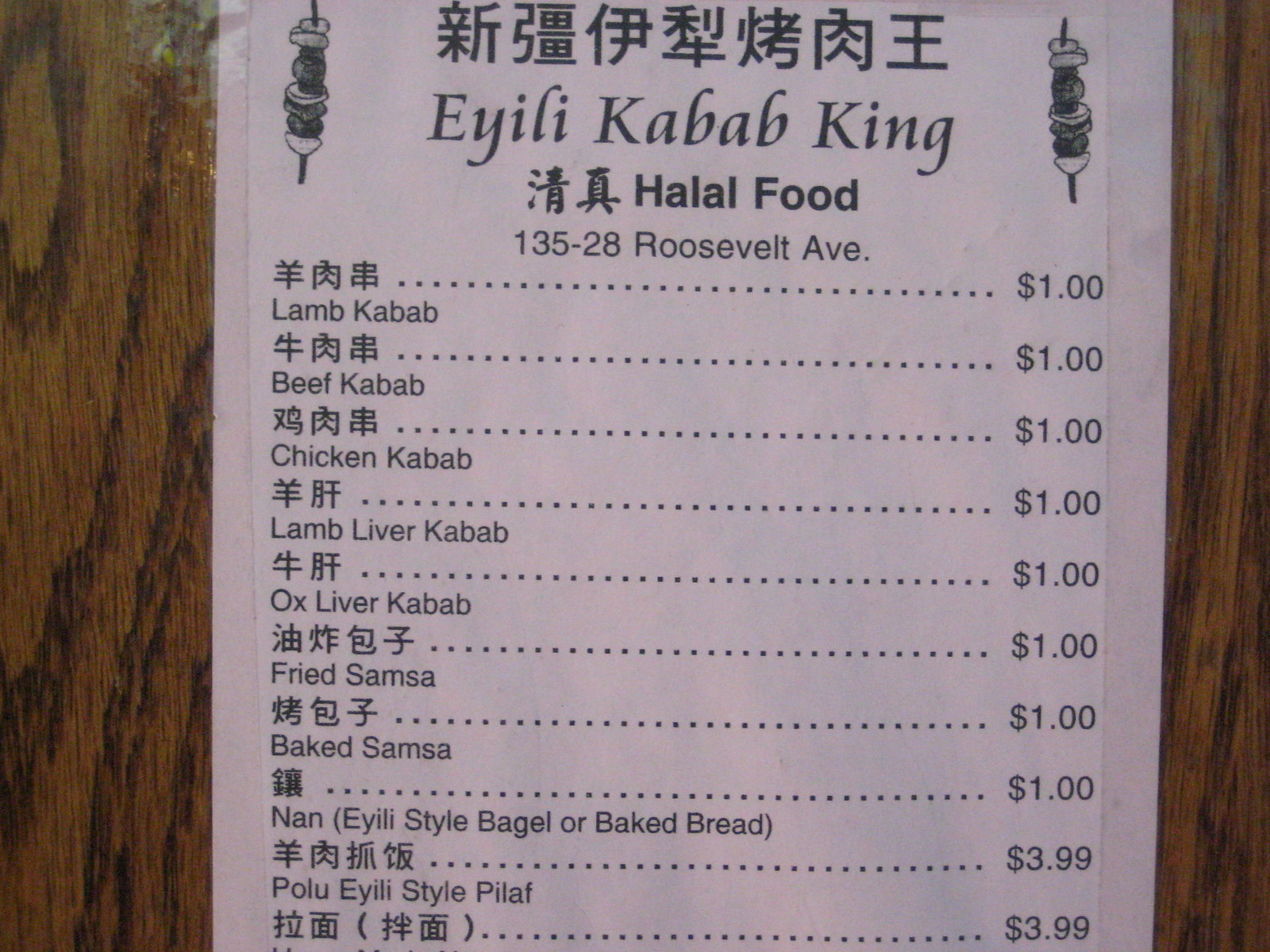This image captures a compact, monochrome menu detailing offerings from a restaurant named "Eylili Kebab King." The menu, smaller than a standard piece of notebook paper, appears to be printed with Asian characters prominently displayed at the top, flanked by illustrated kebabs - skewers with various items, typically meat, depicted on them.

Directly beneath the Asian characters, "Eylili Kebab King" is printed, followed by the phrase "Halal Food" and the address "135-28 Roosevelt Avenue." The primary section of the menu lists an array of kabab options - lamb kebab, beef kebab, and chicken kebab - among others. Traditional dishes such as Samsa, naan, and a type of pilaf are also featured. 

Each dish is accompanied by Asian characters with English translations. The pricing information is located to the right of each item, with most kababs priced at $1.00, while naan and pilaf are priced at $3.99 each. Between the product names and their respective prices, a series of dotted lines provides a clear and organized structure to the menu layout.